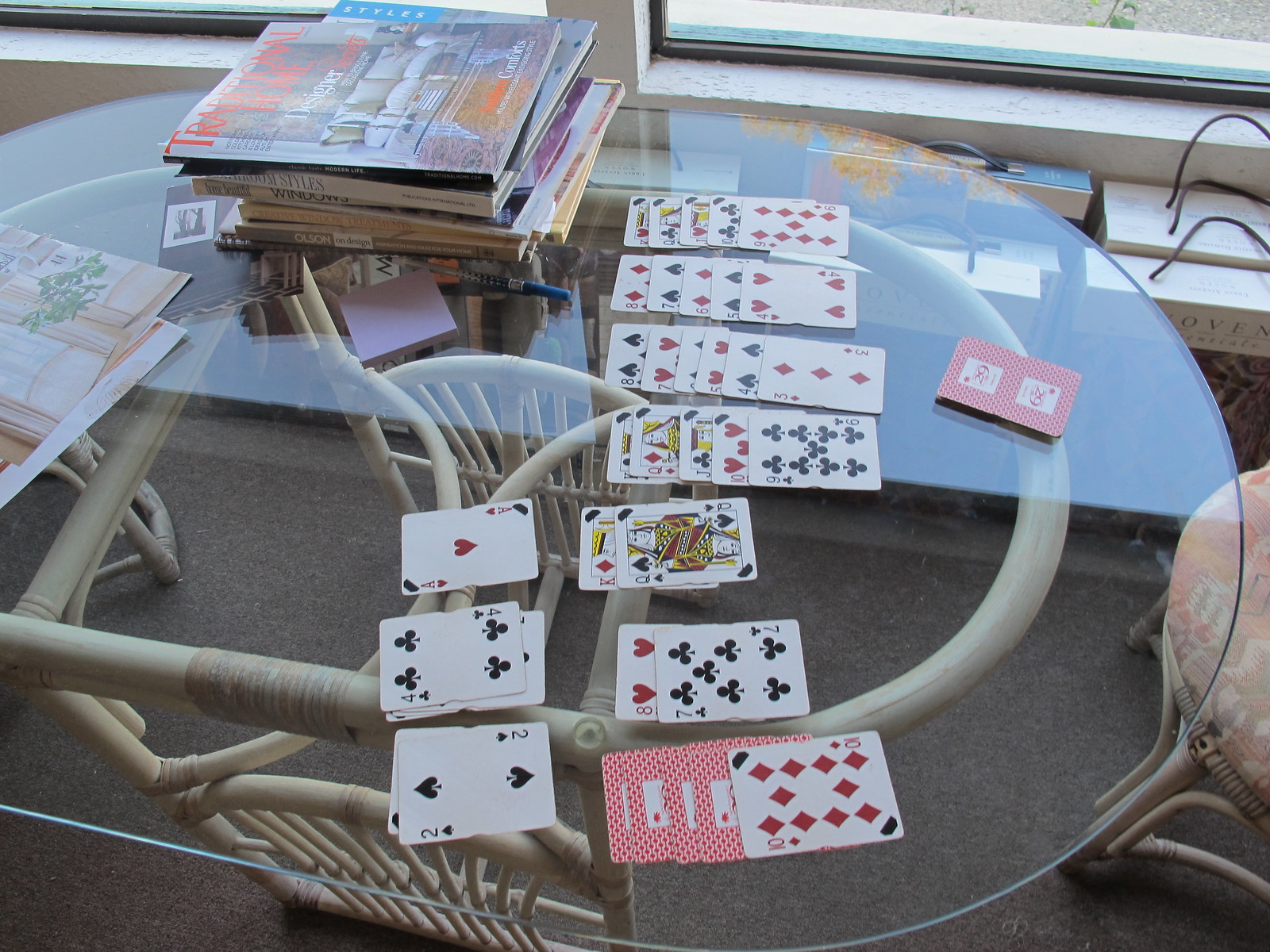The image depicts a glass oblong-shaped table supported by a structure combining metal and a wicker design. On the table, there are various playing cards laid out, suggesting a game of solitaire. On the left side of the table are three piles of cards, while on the right side, there are seven stacks arranged in rows. A single stack of unused cards rests in the middle of the arrangement. Towards the top left corner of the table, a stack of books is neatly placed. The table is positioned near a window with a white windowsill. In the background, there is a wicker chair with a light beige cushion that appears well-worn.